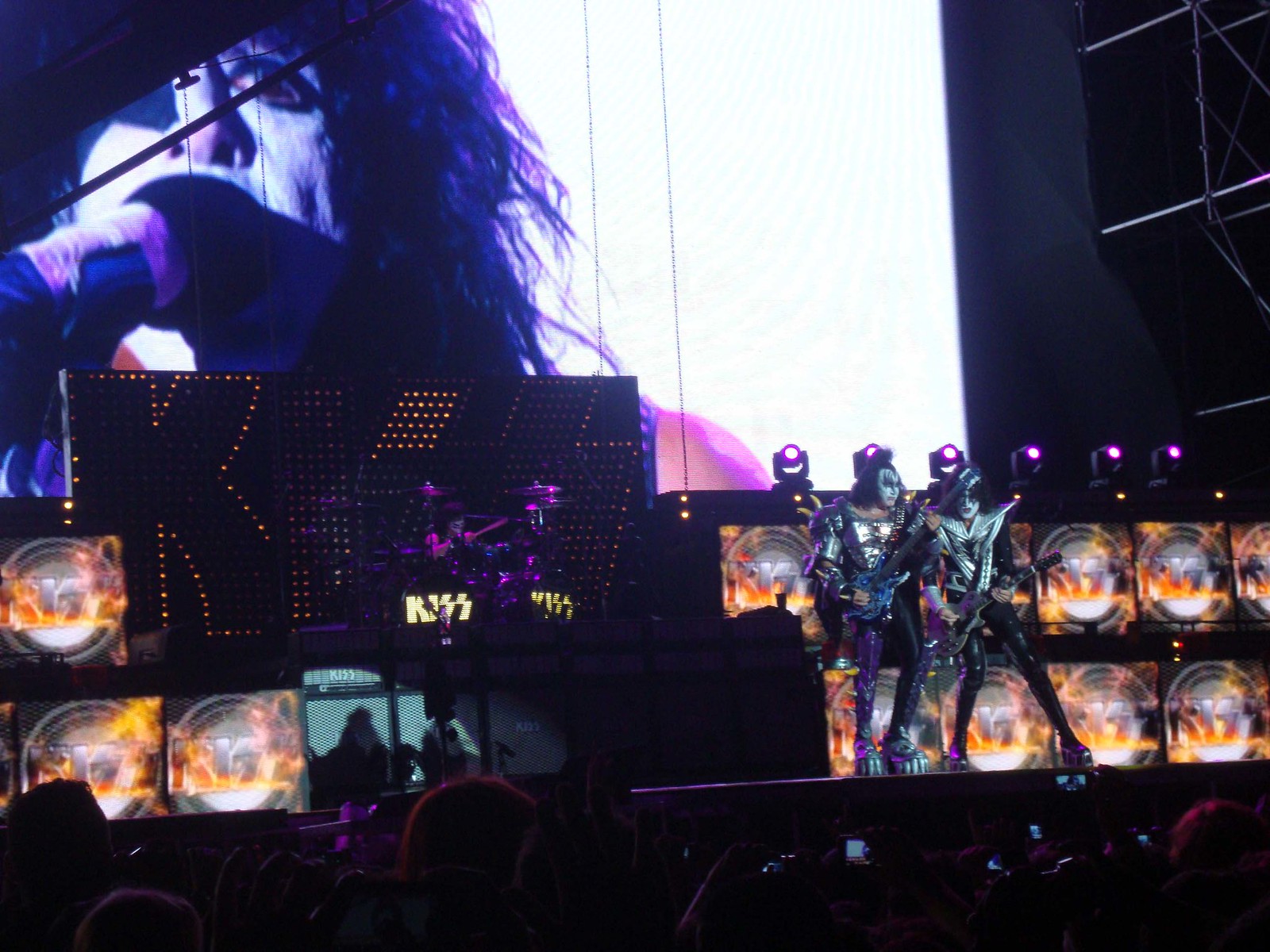This rectangular photograph, wider than it is tall, captures the electrifying atmosphere of a KISS concert. Dominating the left side of the image is a large black banner with the iconic "KISS" logo outlined in yellow lights. Above the banner, there's a close-up projection of a singer, likely Paul Stanley, with long black hair and classic KISS face paint, singing into a microphone against a bright white background.

On the stage, towards the right side, stand two band members—one appears to be Gene Simmons, identifiable by his distinctive makeup. Both are donned in signature KISS costumes, featuring leather pants, space-themed tops, and elaborate footwear. The performers hold guitars, adding to the dynamic energy of the scene.

The stage is bathed in an array of purple hues, with intricate lighting systems and big spotlights enhancing the visual spectacle. Behind the performers, there's a massive screen displaying close-up images of the band, ensuring that even the members of the audience farthest from the stage can see the performers up close.

At the bottom of the image, the silhouettes of the crowd are faintly visible, with some people holding up their phones to record the electrifying performance. Despite the dark lower corners of the photograph, the energy and excitement of the concert are palpable, making this a vivid visual document of a live KISS performance.